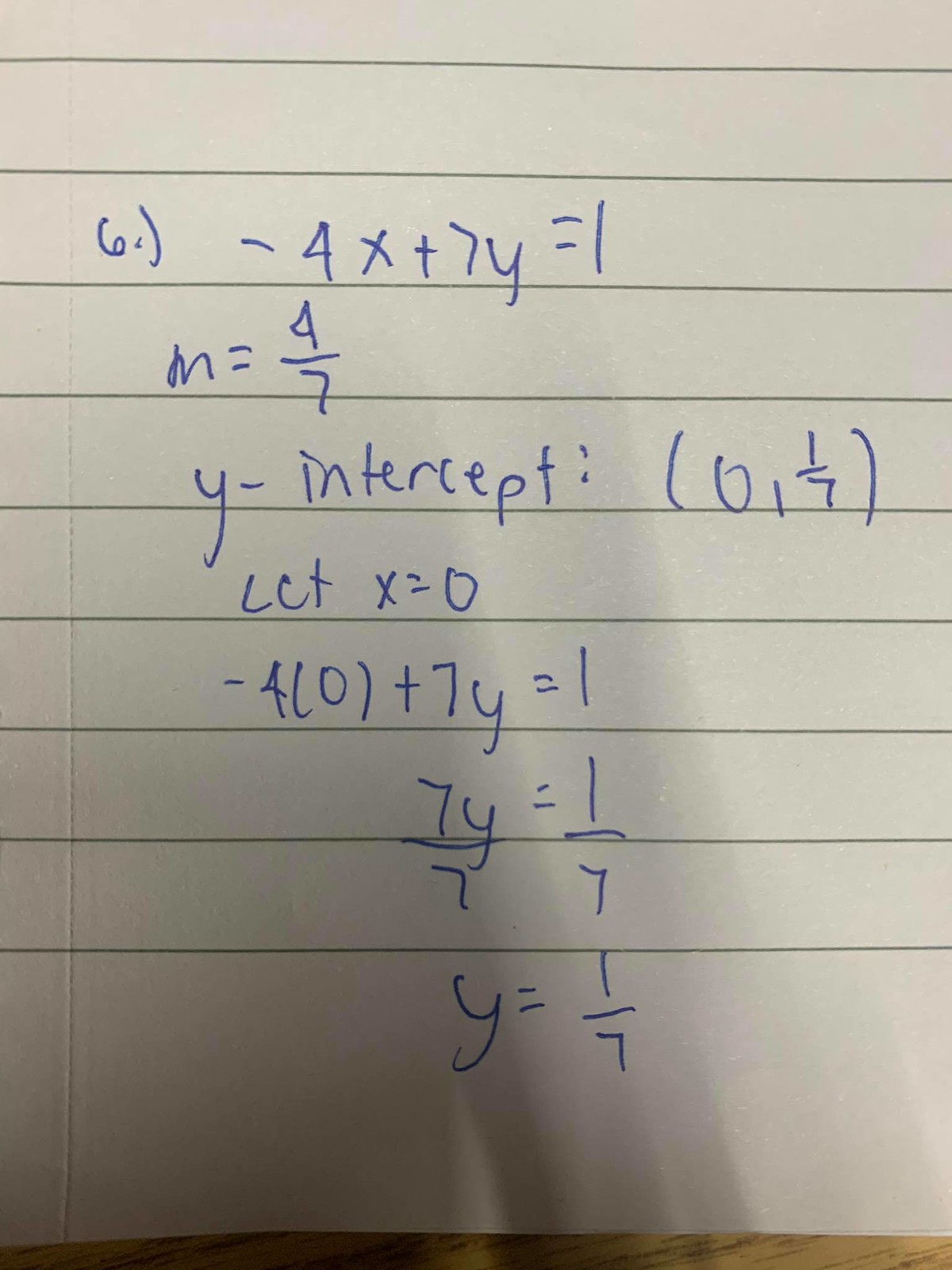This is a detailed description of a photograph depicting a piece of ruled paper. The paper features light gray lines that are fairly widely spaced. On the left side of the sheet, there is a white line or possibly a raised area indicating the margin. The background of the image includes a small portion of wood grain, suggesting that the paper is placed on a wooden surface.

The main focus of the image is a handwritten mathematical equation situated near the bottom of the paper. The equation reads:

```
6.
...
( - 4 x + 7 y = 1
m = (4 / 7 y) - intercept: (6, 1.7)
LCT X = 0
- 4 (0) + 7 y = 1
7 y / 7 = 1 / 7
y = 1 / 7
```

The handwriting indicates that this is problem number six on the paper, likely part of a set of math problems, potentially encompassing algebra or another branch of mathematics.